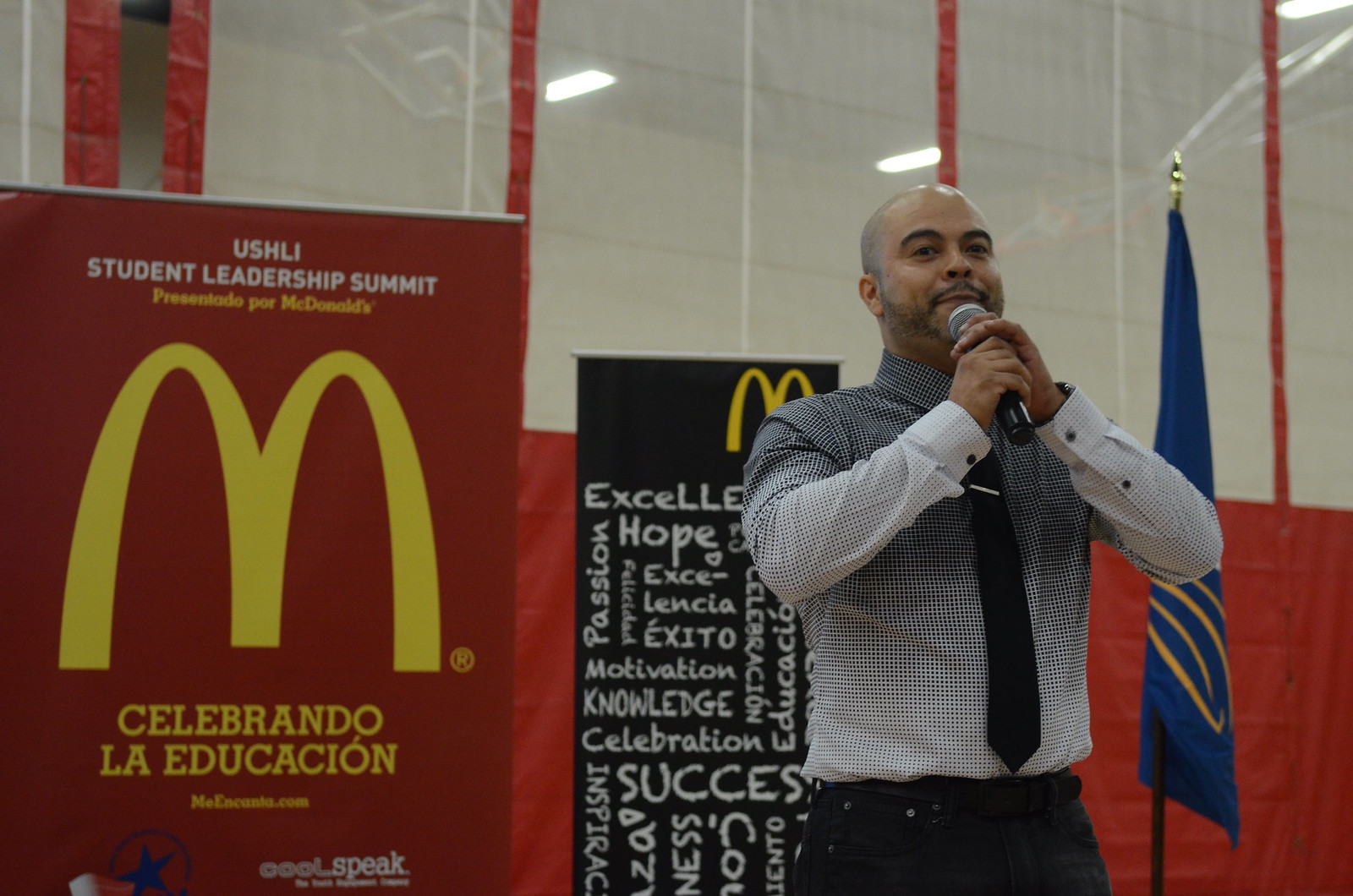The photograph captures a bald, lightly bearded man with a mustache, standing in an indoor setting and giving a presentation. He’s holding a microphone with both hands and is dressed in a dress shirt with a fine black and white checkered pattern that gives it a dark gray appearance, paired with a black tie and black pants. The man is standing in front of two signs adorned with the McDonald's logo. One red sign, featuring Spanish text, reads "US HLI Student Leadership Summit presentado por McDonald's Celebrando la educación," suggesting an educational conference or summit. The other sign, in black, displays a word cloud including words like "excellence," "success," "knowledge," and "motivation," likely meant to inspire the attendees. The background features a predominantly red backdrop, a blue flag with a yellow design, and a semi-transparent white netting. His slight smile and poised stance suggest he is confidently leading the presentation.